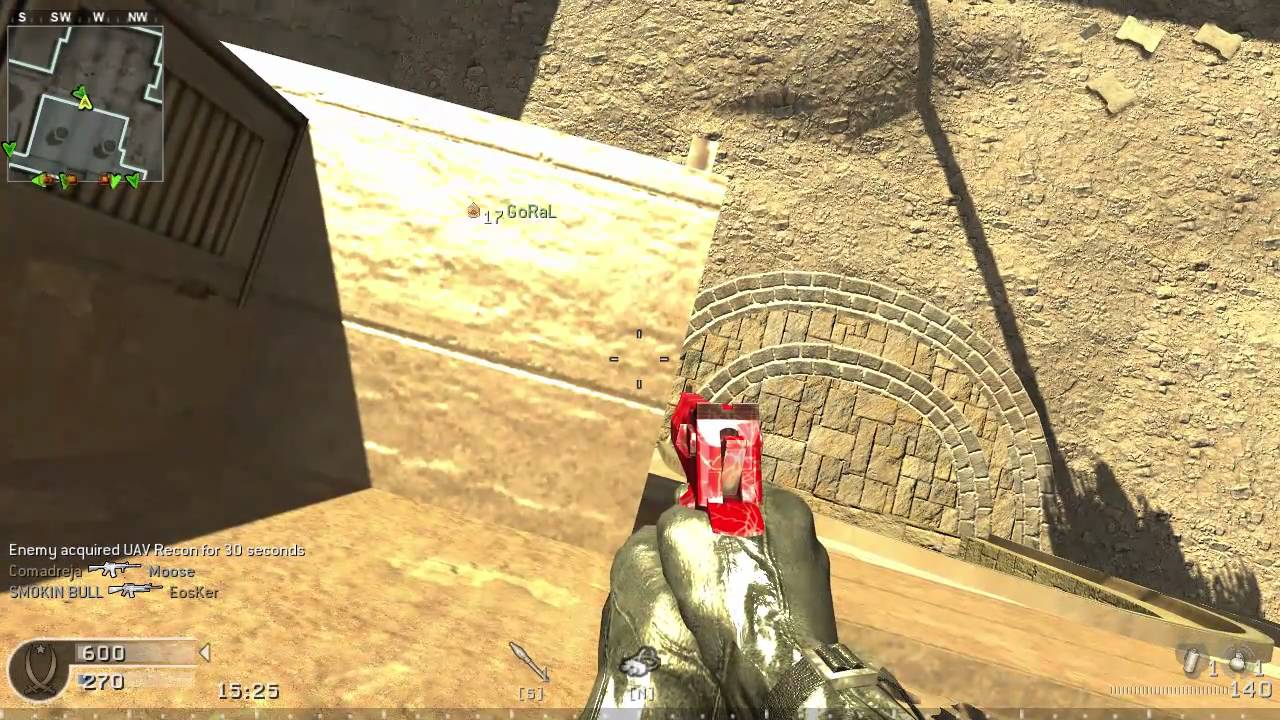The image is a screenshot from the first-person shooter game Call of Duty. The player character, viewed from a first-person perspective, is seen wearing gloves and aiming a shiny, metallic red pistol downwards from the top of a building. The scene appears to be set in a desolate, war-torn area with a cobblestone sidewalk and scattered loose bricks, surrounded by dirt, enhancing the atmosphere of destruction. In the Heads-Up Display (HUD), located at the bottom of the screen, detailed information includes the player's points, time left in the match, and the inventory of grenades and flash grenades. The player's health status is also visible. Additionally, in the upper left corner, a minimap displays the layout of the area and the player’s current location, contributing to the tactical gameplay experience.